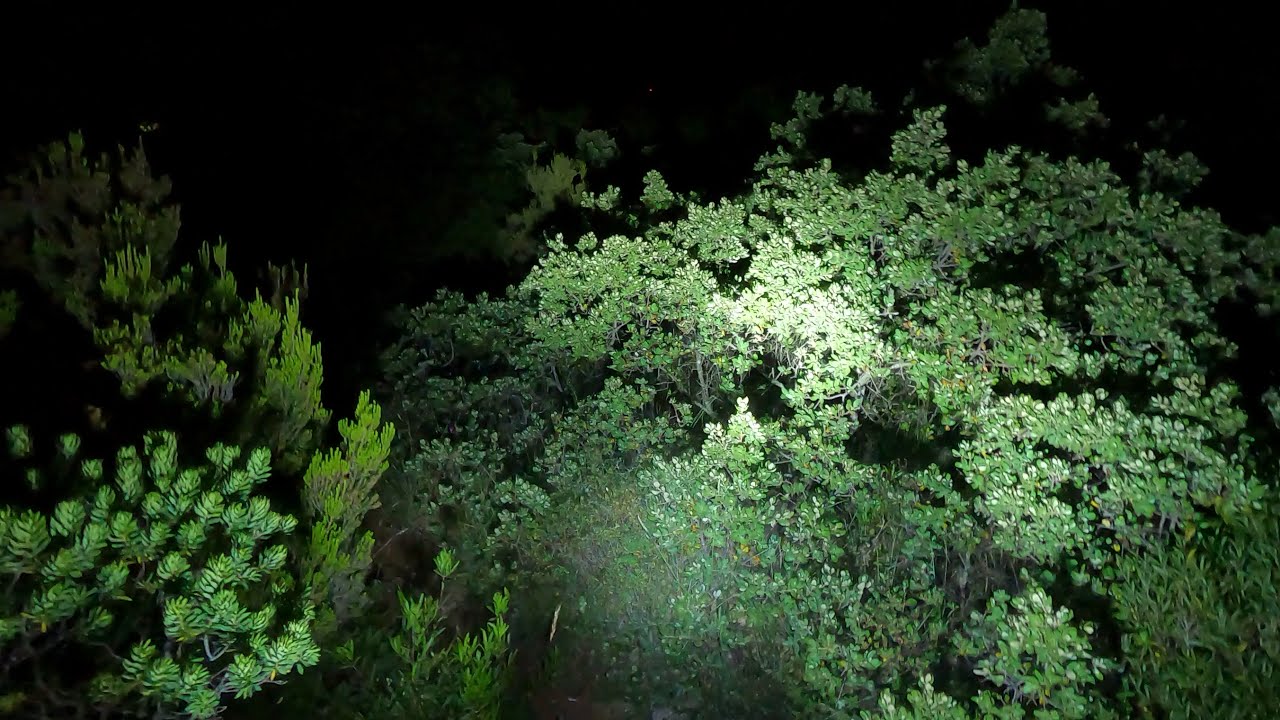The photograph captures a serene outdoor scene at night, presented in full color and framed horizontally. The image showcases a variety of lush, green foliage, predominantly trees and shrubs, brightly illuminated by a large flashlight or spotlight set against a pitch-black background. This strong artificial light highlights the different shades of green, from deep emerald to yellowish tones, and reveals the intricate details of the leaves and branches. The vegetation appears healthy and vibrant, indicative of a warm summer night, with no signs of seasonal change or decay. There are no people, animals, or text present in the image, making it a pure, focused depiction of nighttime nature bathed in the stark contrast of darkness and light.